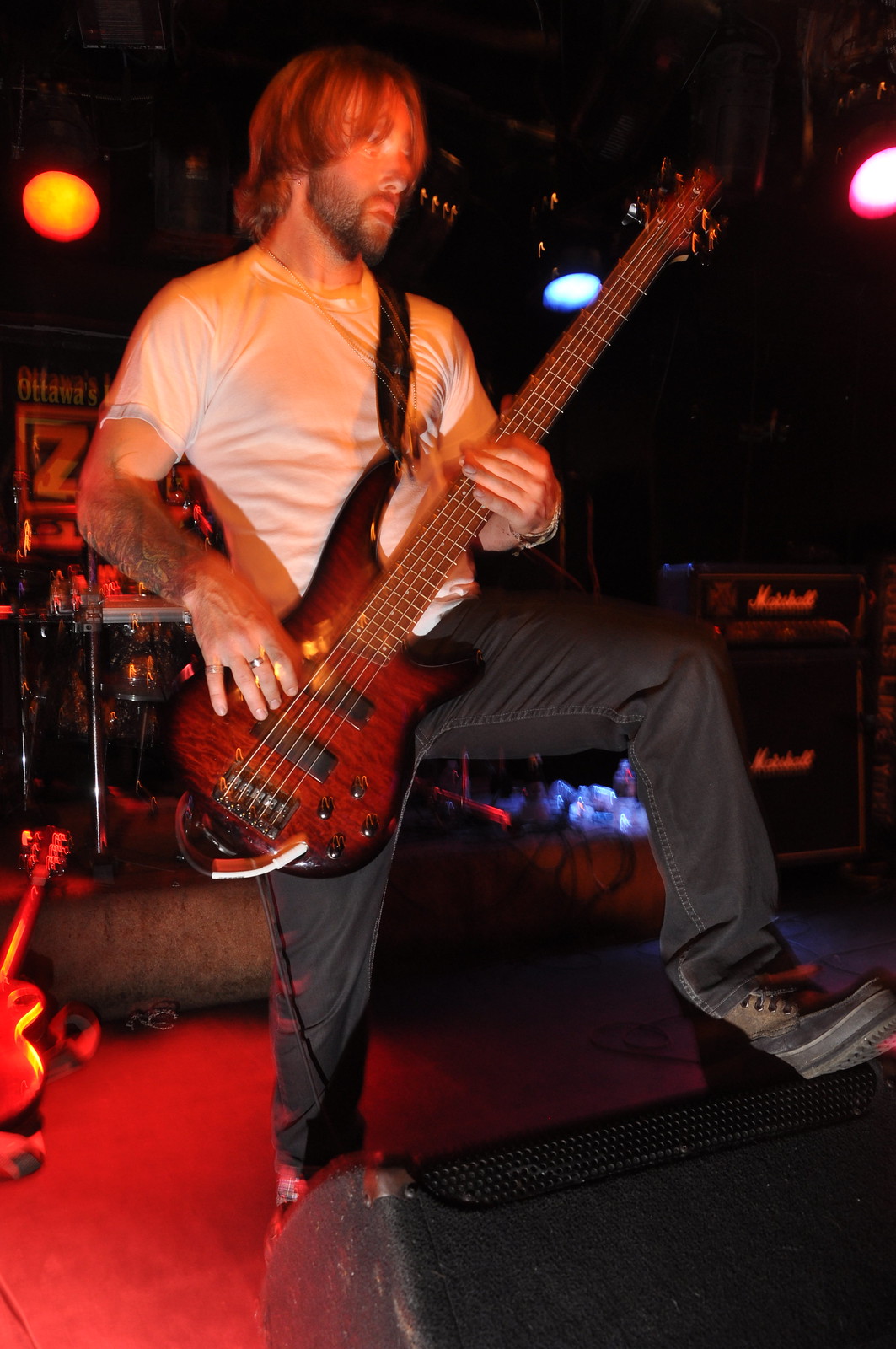In this photograph, we see a man performing live at a music club. He has his left foot perched on a monitor speaker at the front of the stage, striking a dynamic pose. The man, adorned with a tattoo on his right arm, is playing an electric guitar with a body that appears to be of burnt orange or brown wood. His attire includes a white t-shirt and black jeans, and he is wearing sneakers. He has somewhat long, shaggy blondish-brown hair that covers his ears, and a short-cropped beard. Behind him, there’s a dark wooden floor, a drum set with black shells and white drumheads, and another guitar leaning against a part of the stage. Also visible are two large Marshall amplifiers to the right. The club's signage, partially obscured by the man, suggests the name "Ottawa's." Above him, several colored lights illuminate the scene, including orange, blue, and pink ones, enhancing the vibrant atmosphere of the music club.